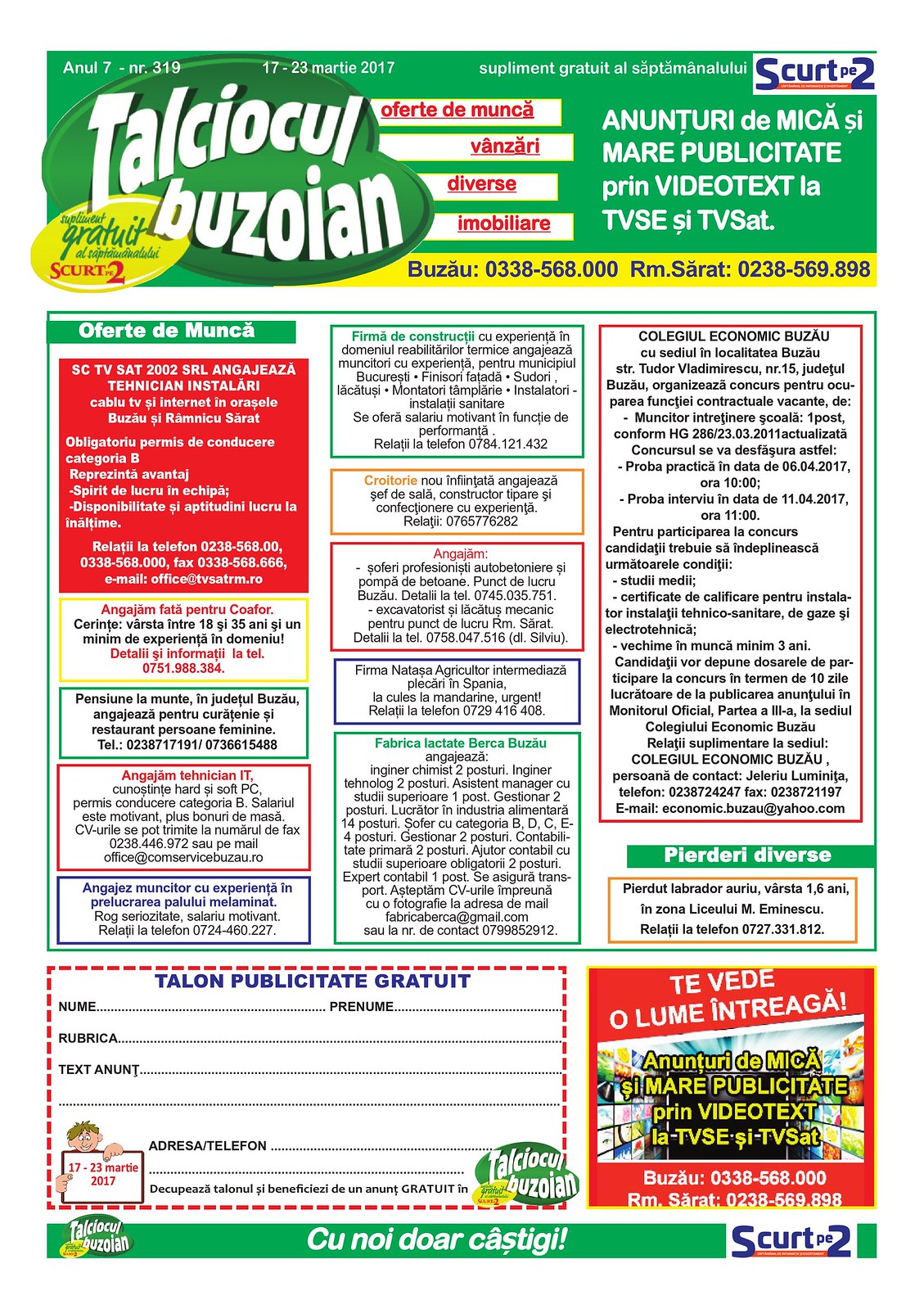This image appears to be a section from an international newspaper or magazine, likely from the social section, and is written in a foreign language, possibly Spanish, Mexican, or Italian. The layout is predominantly green and white with both red and white script. The content is organized into squared-off sections that contain various details, including offers and advertisements for different services, possibly including a category for real estate based on the term "immobiliary." Telephone numbers are prominently featured within these offers, suggesting they are small advertisements or classifieds. At the very bottom, there is a distinct section that seems to resemble a coupon or a subscription form, with the phrase "TALON PUBLICAT GRATUIT" followed by fields for personal information like "NUM," "PRENUM," "RUBRICA TEXTA," and "ADDRESSE TELEPHONE." This final section hints that readers may be able to send in the form for a free subscription or offer.